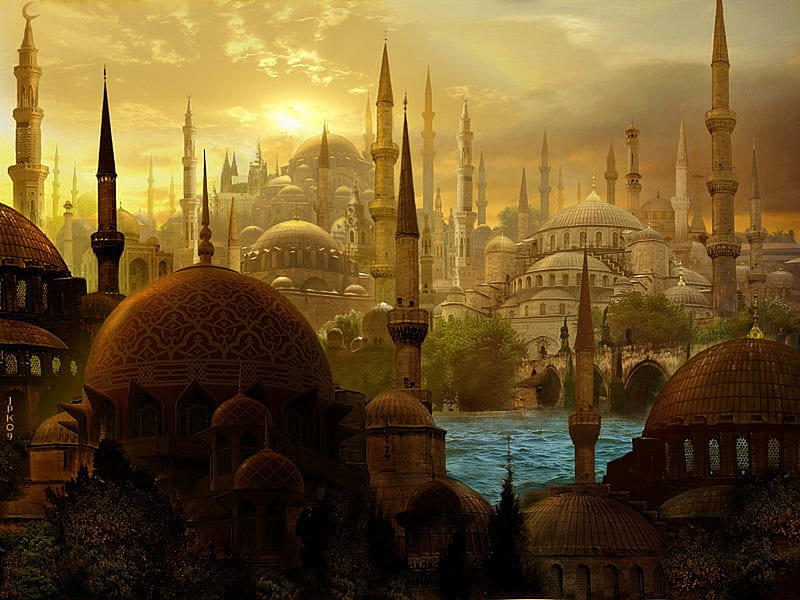The image depicts a meticulously crafted, either painted or computer-generated, depiction of a fantastical city, full of intricate architectural details. Dominating the foreground are several dark brown buildings, characterized by domed, semi-hemisphere roofs, many topped with pointy spires or steeples. Just beyond these structures lies a choppy, turquoise river or canal, its unsettled waters suggesting a windy day. A bridge arches over this waterway, reminiscent of the ones spanning the River Seine in Paris, complete with openings for water flow. 

On the far side of the river, a multitude of similarly styled buildings extend into the distance, their domes and cylindrical towers creating a cityscape dotted with dozens of spires and steeples. The structures appear lit by a setting or perhaps rising sun, casting a warm yellow glow across the scene. The sky above is a mix of light clouds tinged with sunlight and darker clouds moving in from the right, providing a dramatic backdrop. The overall horizontal rectangular composition of the image presents a harmonious blend of historical and fantastical elements, evoking a sense of wonder and timelessness.